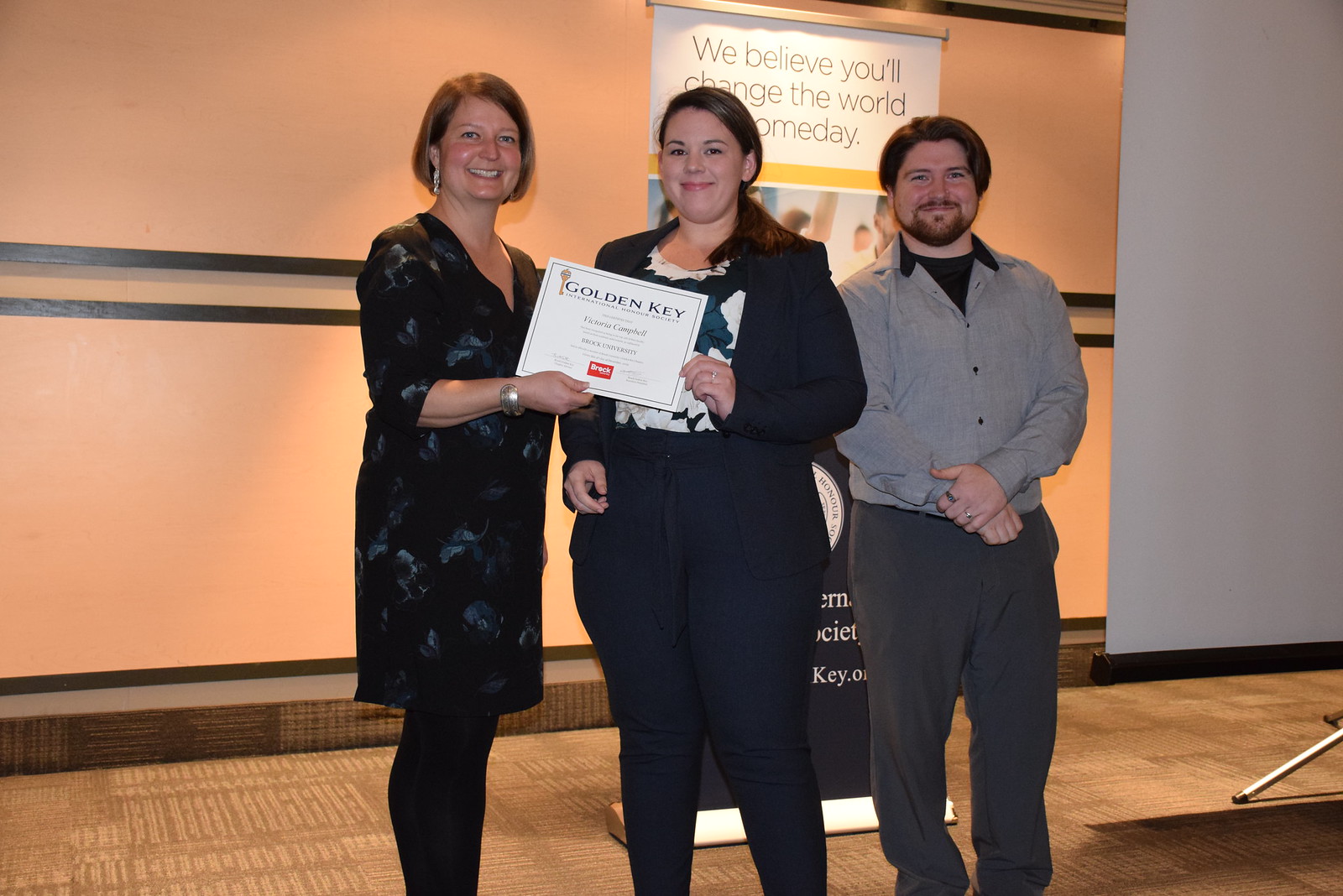In a brightly lit function hall with a beige wall intersected by black horizontal lines and a partially visible banner reading "We believe you'll change the world someday," three smiling individuals are captured during an award presentation. The scene takes place in front of a projector screen, currently blank, and on a brown-carpeted floor. On the left stands a middle-aged woman with shoulder-length brown hair and earrings, dressed in a dark-colored, above-the-knee dress adorned with blue roses, paired with dark tights. She is handing a certificate to a younger woman with black hair tied back in a ponytail, who is donning a dark suit jacket over a multicolored dress shirt in shades of blue, black, and white, along with black trousers. The certificate, inscribed with "Golden Key International Honour Society" and the name "Victoria Campbell," is being jointly held by both women. To the right stands a young man with mid-length brown hair and a neatly trimmed beard and mustache, dressed in a grey shirt over a black t-shirt and grey trousers, with his arms crossed. The trio exudes a sense of accomplishment and celebration as they pose for the camera.